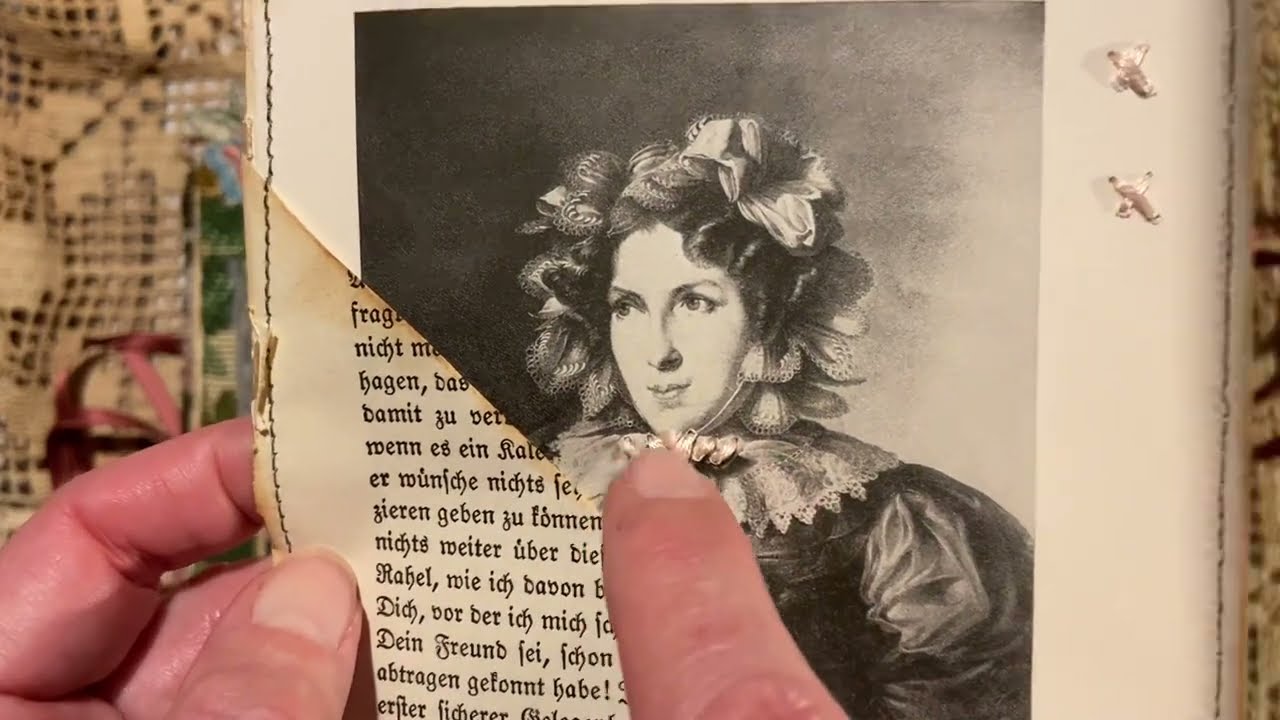The image depicts a detailed scene involving a person holding an old book. The book is gripped by two hands with short, plain nails and lighter-colored skin. The left hand holds the book steadily, while the right index finger points towards the focal point of the image—a black and white illustration of an older woman. Her face is positioned directly at the center of the page, which takes up the entirety of the image. The woman in the illustration has dark, curled hair adorned with a flower and feathers on the left side. She wears an old-fashioned, puffy silk dress with a frilly chiffon collar. Her expression is composed, with dark eyebrows and lips gently pursed as she gazes off to the right. There is a noticeable diagonal cut across the illustration which does not hinder the visibility of her face but obscures her right shoulder down while showcasing her left shoulder down to her waist. The background contains a mix of colors including shades of gray, pink, purple, green, light blue, and tan. In the bottom left-hand corner, there is text written in a foreign language, adding to the sense of a historical or cultural context. The setting appears to be indoors, possibly taken inside someone's home.